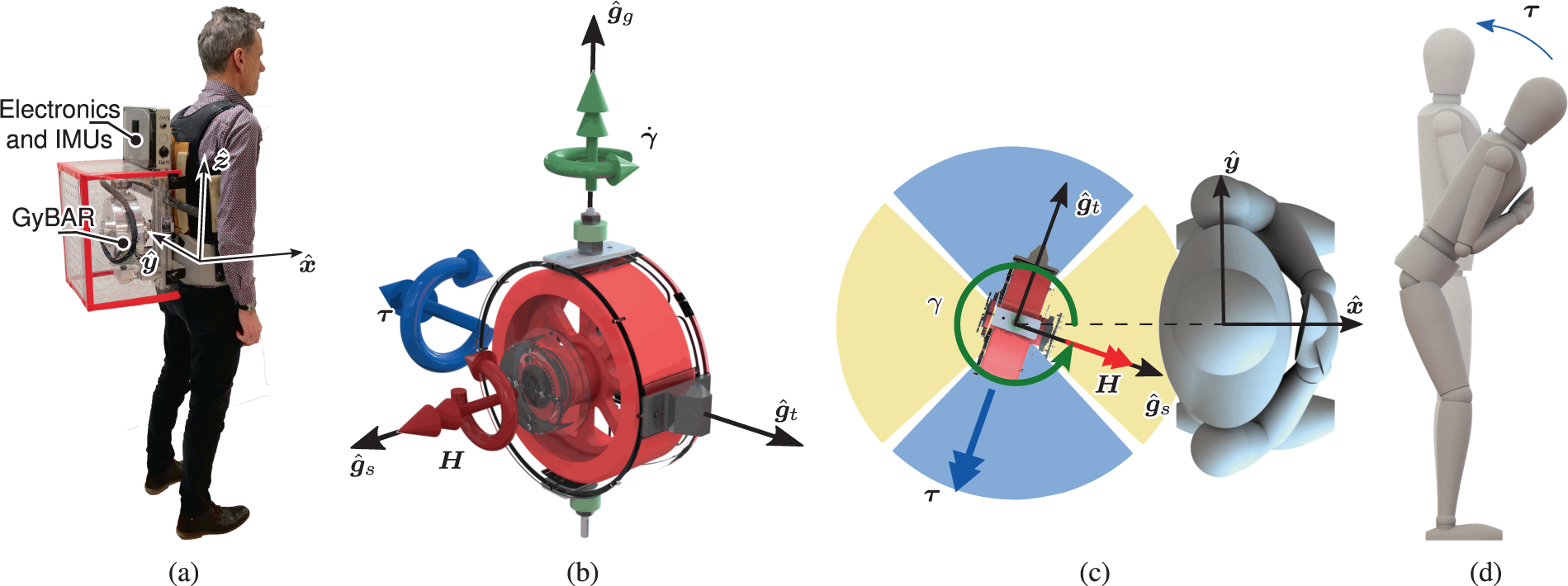The image is a comprehensive educational diagram illustrating a prototype device strapped to a person's back, depicted through four labeled figures (A, B, C, and D). Figure A introduces the device equipped with electronics and IMUs, highlighting directional axes (Y, X, Z) and specific components like a GY bar. The subject—a man wearing a button-down shirt, black pants, and black shoes—demonstrates the attachment method, featuring a clear casing with a red metallic frame. Figure B offers a close-up of the internal mechanism, showing a red cylindrical object and three rotational axes marked with green, blue, and red arrows, indicating the IMU's (Inertial Measurement Unit) movement capabilities. Figure C provides a top-down view of the setup, emphasizing the gyroscopic elements and their spatial orientation on the human model. Lastly, Figure D illustrates the functional range of motion, depicting the individual bending forward and returning to an upright position, showcasing the device's dynamic adaptability.